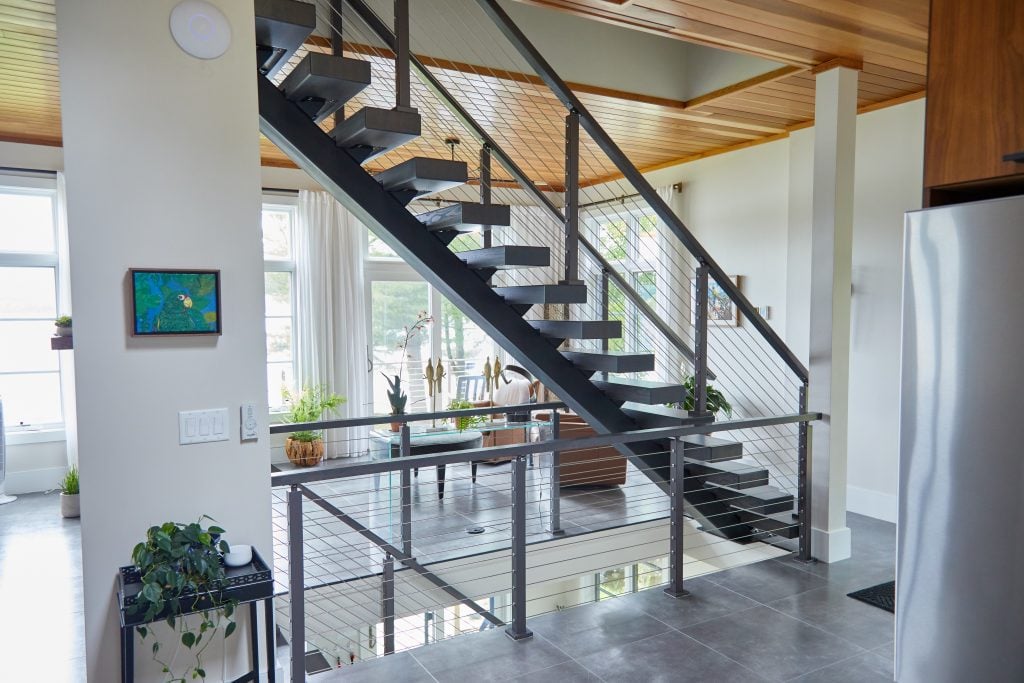The image captures the modern, open interior of a house with a distinct floor plan encompassing multiple levels. A stairway in the middle ascends toward an attic through a small opening in the ceiling, alongside another staircase that potentially leads downstairs. Predominantly white, the room features walls and ceiling panels of finished wood, contrasted by gray tiles on the floor reminiscent of an office building. Large glass windows and doors along the back wall allow natural light to flood the spacious area, with views of trees outside. On the right side, there's what appears to be a refrigerator or a wall, and a thermostat. A white wooden pillar stands near the staircases, beside a small table adorned with an overflowing ivy plant and a blue-themed picture, with a light switch situated between them. The expansive room also contains a small living area setup, enhancing the open-plan aesthetic.